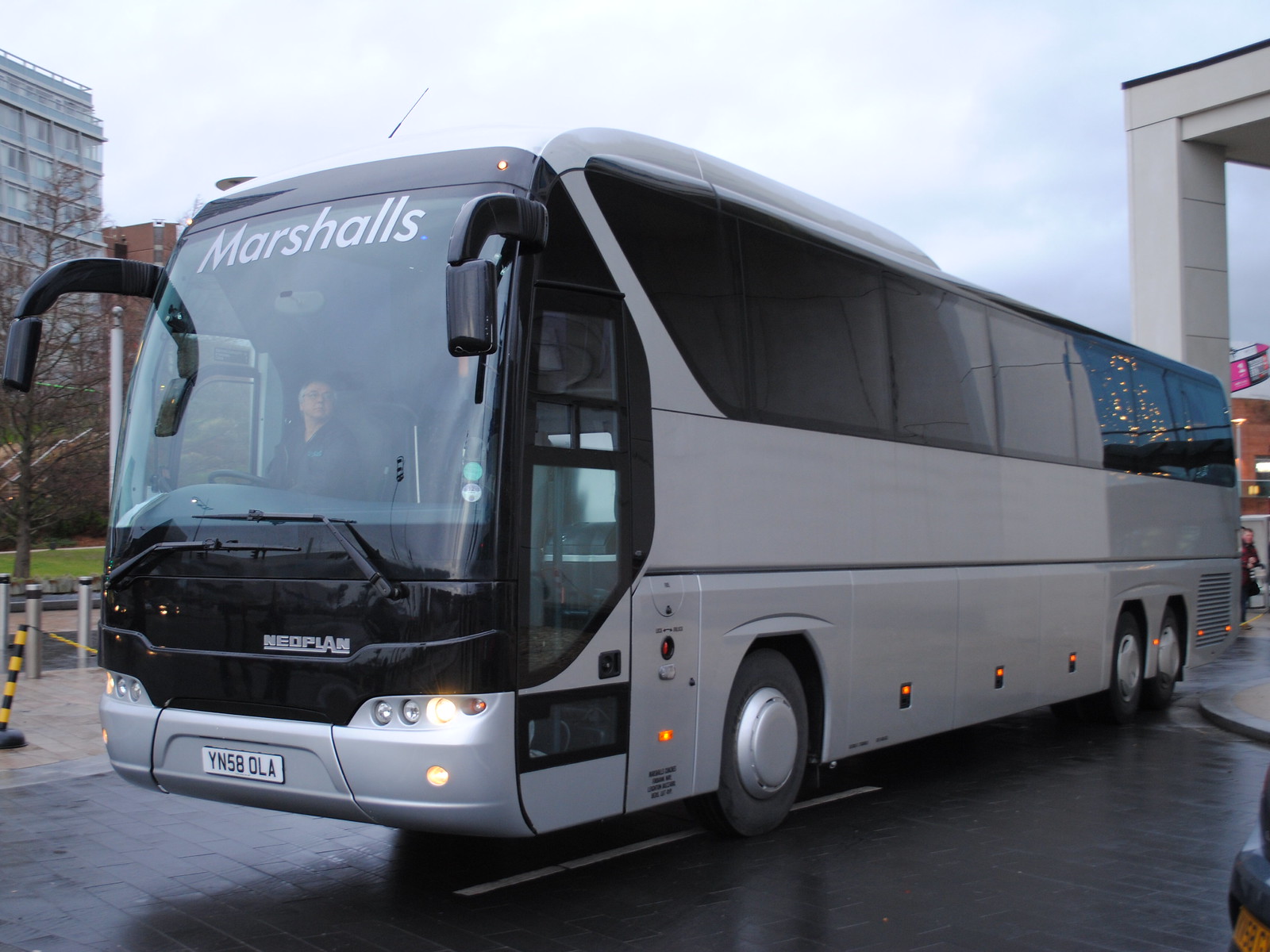This horizontal, rectangular image depicts a sleek, modern, silver bus parked on a dark surface. It features large, tinted black windows along the side, a prominent glass front, and the word "MARSHALLS" inscribed in large letters at the top front. Notably, there is a small badge at the bottom right of the front that reads “Neo Plan,” and the license plate is visible with the number Y-N-5-8-O-L-A.

The bus is centered in the image, with its reflective surface mirroring the visible sky, which is partly clouded, indicating daytime lighting conditions. In the background, on the right side, a partial view of a building, including a pillar and roof, can be seen. The left side features several taller buildings contributing to an urban setting. There are a few people walking around in the vicinity, adding life to the scene.

Inside, one can barely make out the driver situated on the passenger side, indicating the bus is designed for left-lane driving. The sharp and contemporary design of the bus suggests it might be a highly modern passenger vehicle or even a high-end recreational one. The detailed array of colors present—black, white, gray, silver, orange, red, purple, pink, green, and brown—contrasts interestingly with the sleek, silver exterior of the bus.